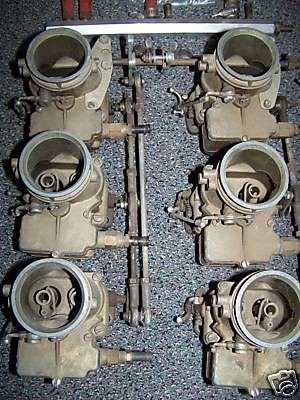The image depicts a color photograph of six identical machine components, possibly engine parts or elements of a transmission, arranged in a neat, orderly fashion. Each component appears to be about eight inches by seven inches, featuring a square base with two round holes, topped by a large circular element. The components are slightly aged with some rust and dirt, indicating their use or age. They are positioned on a surface that could be interpreted as a Corian countertop, tile, or even gravel, characterized by a bluish, purple, and black paisley-like design. Tubes and pipes emerge from the right side of each component, connecting to other parts, hinting at a complex mechanical function. Above these components is a small white shelf with additional red and metal tubing, rounding out the industrial, machine-oriented scene. The photograph is highly detailed, clearly intended to showcase these mechanical parts, possibly for sale or detailed inspection.